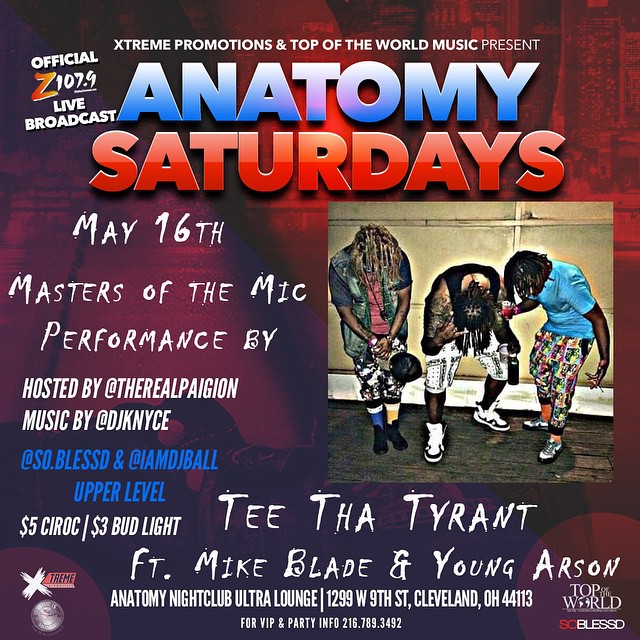The promotional image features a rich, textured design with a bold color scheme and detailed information:

At the top, a vibrant red triangular background blends into a purple backdrop.

In striking blue and red fonts, the text announces: "Extreme Promotions and Top-of-the-World Music Present Anatomy Saturdays."

In white font below, it reads: "Official Z 107.9 Live Broadcast."

Further down, the date "May 16th" is prominently displayed alongside the event details: "Masters of the Mic Performance," and a note that it is "Hosted by @TheRealPaganPageant."

Music for the event will be provided by "@DJKNYC," "@SoBlessed," and "@IAmDJBall."

The caption continues with a special note in blue font: "Upper level - $5, I Rock - $3, By Light - T-Thaw, Tyrant FT Mike Blade, and Young Arson."

The location for the event is specified as "Anatomy Club, Nightclub, Ultra Lounge," followed by the address and a phone number for VIP and party information.

The sides of the image are adorned with the words "Extreme" on the left and "Arson Top-of-the-World" on the right, along with "See Blessed."

In the central part of the image, there is a dynamic picture of three people dancing energetically. They are bent over slightly as they move on the dance floor, wearing stylish sneakers and sporting braided hair.

This image is vibrantly designed to capture attention and provide all necessary details for the upcoming event at Anatomy Saturdays, promising an exciting night filled with music and performances.